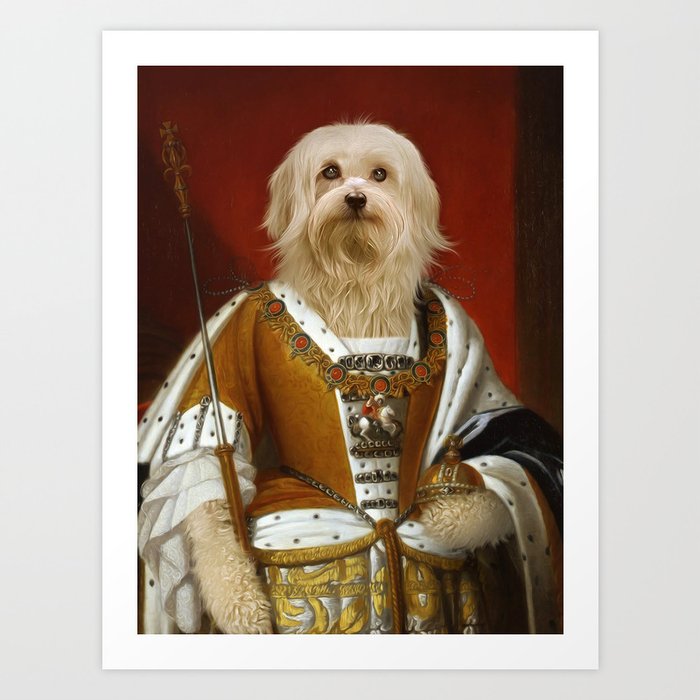The image is a vertical-oriented portrait of a regal-looking dog, which appears to be either a Maltese or a Yorkie, adorned in lavish, royal attire. The dog's long, white fur is prominently displayed, adding to its majestic appearance. This satire image humorously replaces a human royal figure with a dog, creating a whimsical depiction of aristocratic elegance.

The dog is dressed in an elaborate white and brown robe, decorated with intricate designs and lace around the edges of the shoulders. A chain adorns the neck and chest area, enhancing the imperial look. The pose is dignified, with the dog holding a metallic ball, possibly a scepter, in its left paw, and a long rod in its right paw, evoking the traditional symbols of royalty. The background is a deep red, contrasting sharply with the attire and elevating the overall regal theme of the portrait.

The image is framed with a light grey matting about two inches wide, providing a sophisticated outer edge. Inside, the portrait itself is bordered by white, further focusing attention on the dignified subject at its center. The setting is brightly lit, ensuring that every detail of the dog’s noble attire and expression is clearly visible.